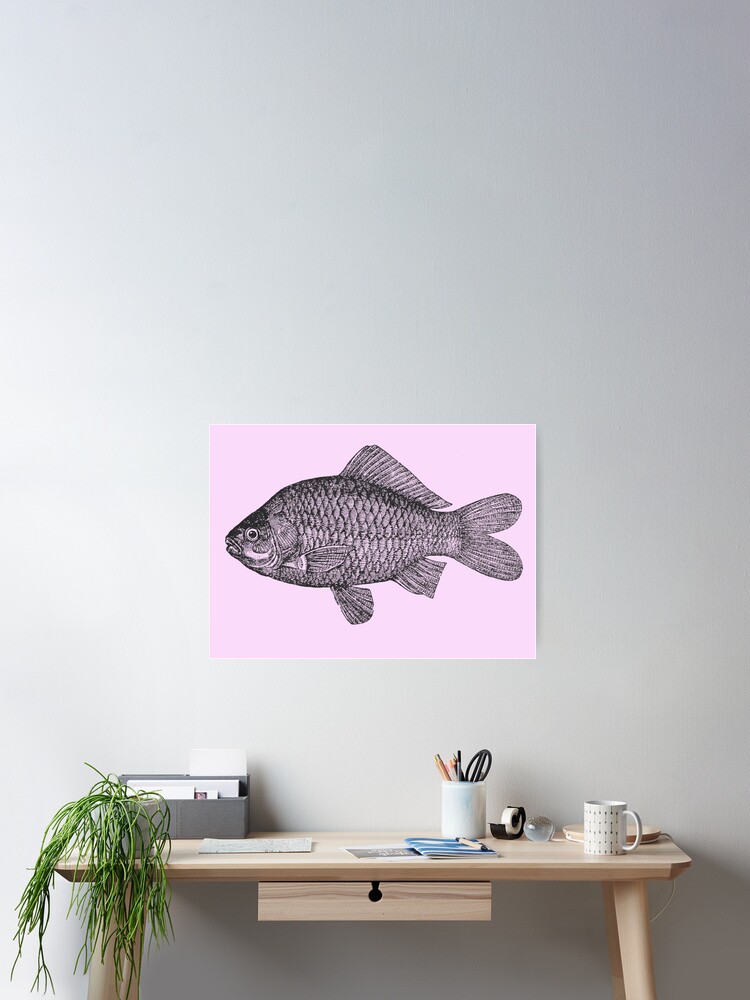The image showcases a detailed sketch of a black fish drawn in pencil, positioned centrally on a carnation pink piece of paper, which hangs horizontally on a white wall. Below the pink paper, a light brown wooden desk occupies the foreground. The desk features a simple design with four legs and a central drawer, which lacks a handle but is marked by an upside-down keyhole-shaped black spot. 

To the left of the desk, a creeping vine-type plant cascades over the side, partially obscuring its white pot. A gray box sits behind the plant, holding a few small papers, with another small paper placed in front of it. In the center of the desk lies a small, folded piece of paper or journal with a tan pen resting on top. 

A white coffee-cup-type mug, filled with various pens, pencils, and a pair of black-handled scissors, is positioned to the right of the journal. Next to it is a roll of scotch tape, and further to the right is a slightly opaque gray bowl, the purpose of which is unclear due to its size. A white coffee mug with an indistinct black pattern appears in the lower-right corner of the desk. 

On the far right side stands a small lamp with a cylindrical white lampshade, a white articulating arm, and a light brown base, completing the array of items arranged neatly on the desk.